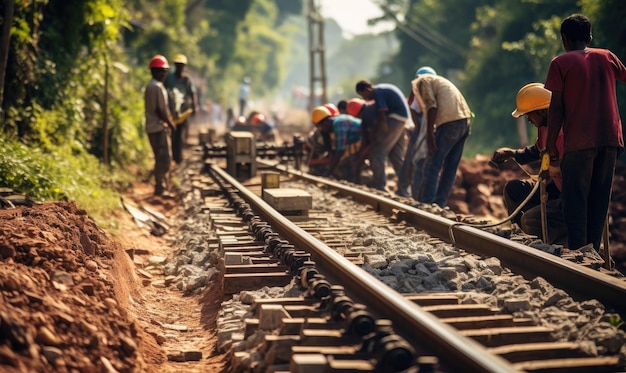The photograph captures an active railway construction or maintenance scene, teeming with around 15 to 20 workers, with more visible in the distance. The setting appears to be in a rural or semi-forested area, possibly in South America, judging by the surroundings and workers. The railroad stretches from the foreground, flanked by dirt and greenery, into the distant horizon, emphasizing the depth and scale of the worksite. The laborers, most donning safety helmets, are busily engaged with various specialized tools and an indistinct crane-like apparatus. These workers are fixing the steel rails to wooden cross ties amidst a gravel-strewn track, surrounded by lush bushes and trees under a bright sunny sky, highlighting the lively spring or summer atmosphere. A large tower stands in the background, adding to the sense of industrial activity and progress.